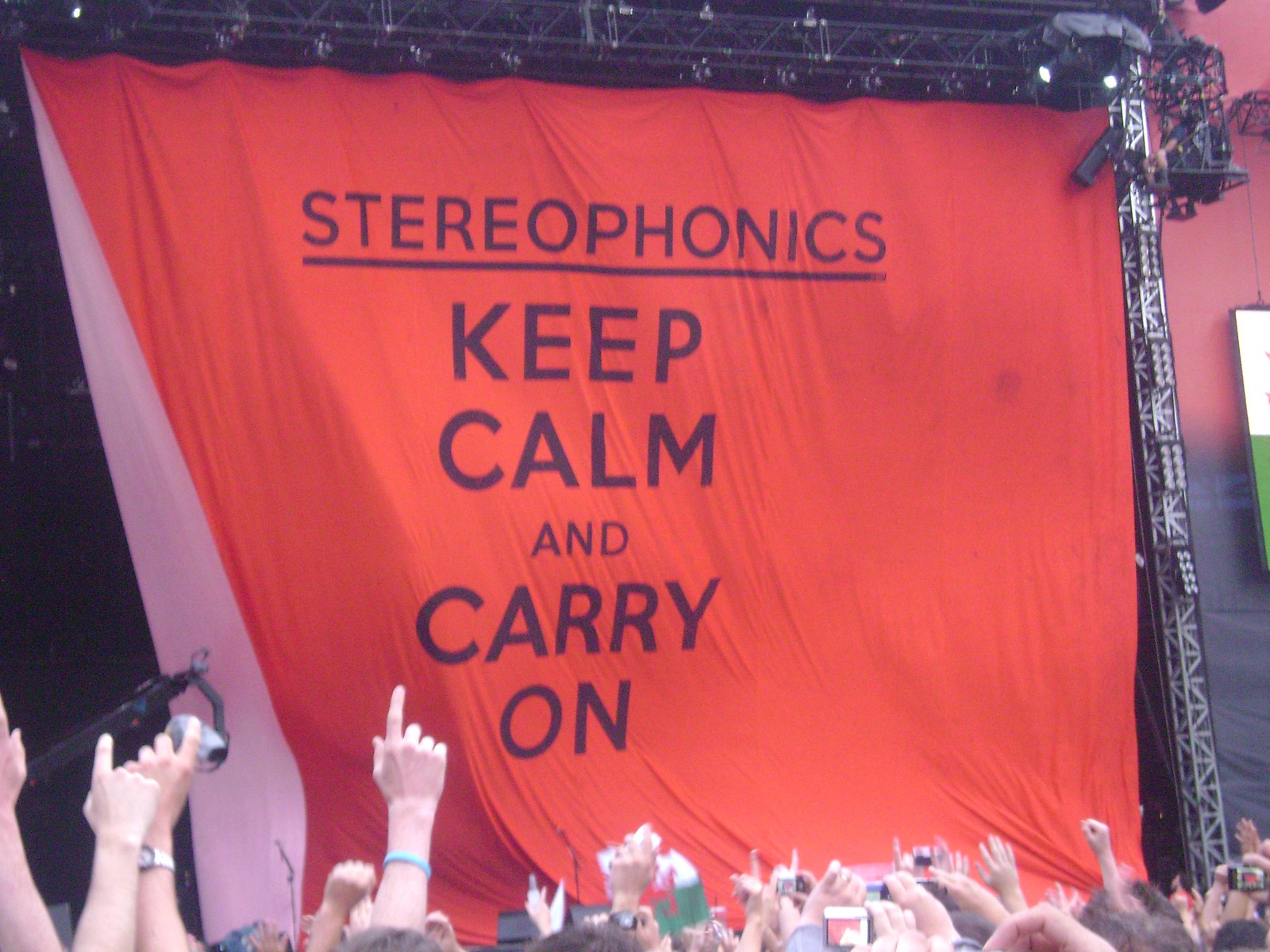The image captures the vibrant atmosphere of a Stereophonics concert, with a solid red curtain bearing the bold text "STEREOPHONICS" in capital letters, underlined, followed by "Keep Calm and Carry On," each word on its own line in slightly smaller text. The scene sets us several rows from the stage, amongst a sea of enthusiastic fans, many of whom have their hands raised – some even holding up one finger. The stage's metal frame, adorned with lights, outlines the background. Attendees are dressed in short sleeves, hinting at a warm, likely outdoor setting, possibly a festival. A particular audience member stands out with both hands raised, holding a camera or other electronic device, ready to capture the moment.